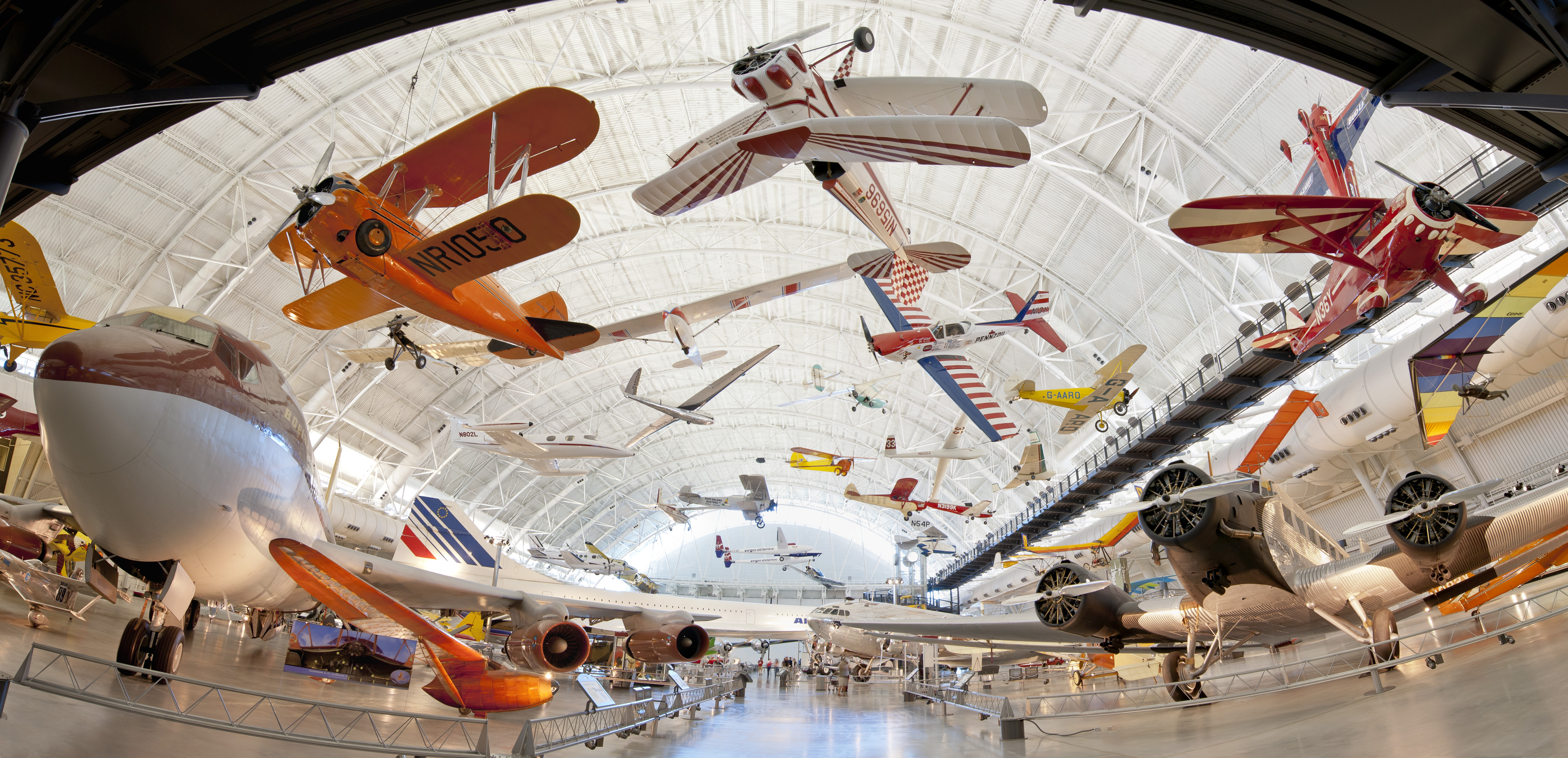This detailed photograph captures the interior of a large, dome-shaped airplane hangar that appears to function as a museum or exhibit space. The fisheye lens creates a curved effect, making the expansive room feel even more grandiose. The ceiling is bright white with a black border, while the shiny concrete floor reflects the abundant light. The scene is populated with numerous old-fashioned, colorful propeller planes, reminiscent of the 1930s and 1940s, often associated with World War I. Many planes are arranged on the ground, safeguarded by safety barriers, while others are suspended from the ceiling, giving the impression of being in mid-flight.

Prominent among the grounded planes, one on the left side is vividly painted in white, red, and yellow. Suspended above and attracting considerable attention are three planes: an entirely orange one on the far left, another white with red stripes in the center, and a red one with white details on the right. Additionally, there's an evocative plane that features an American flag design, hanging among the other airborne displays. Altogether, the hangar contains a dazzling variety of aircraft with diverse designs and color schemes, creating a captivating and nostalgic atmosphere throughout the immense space.